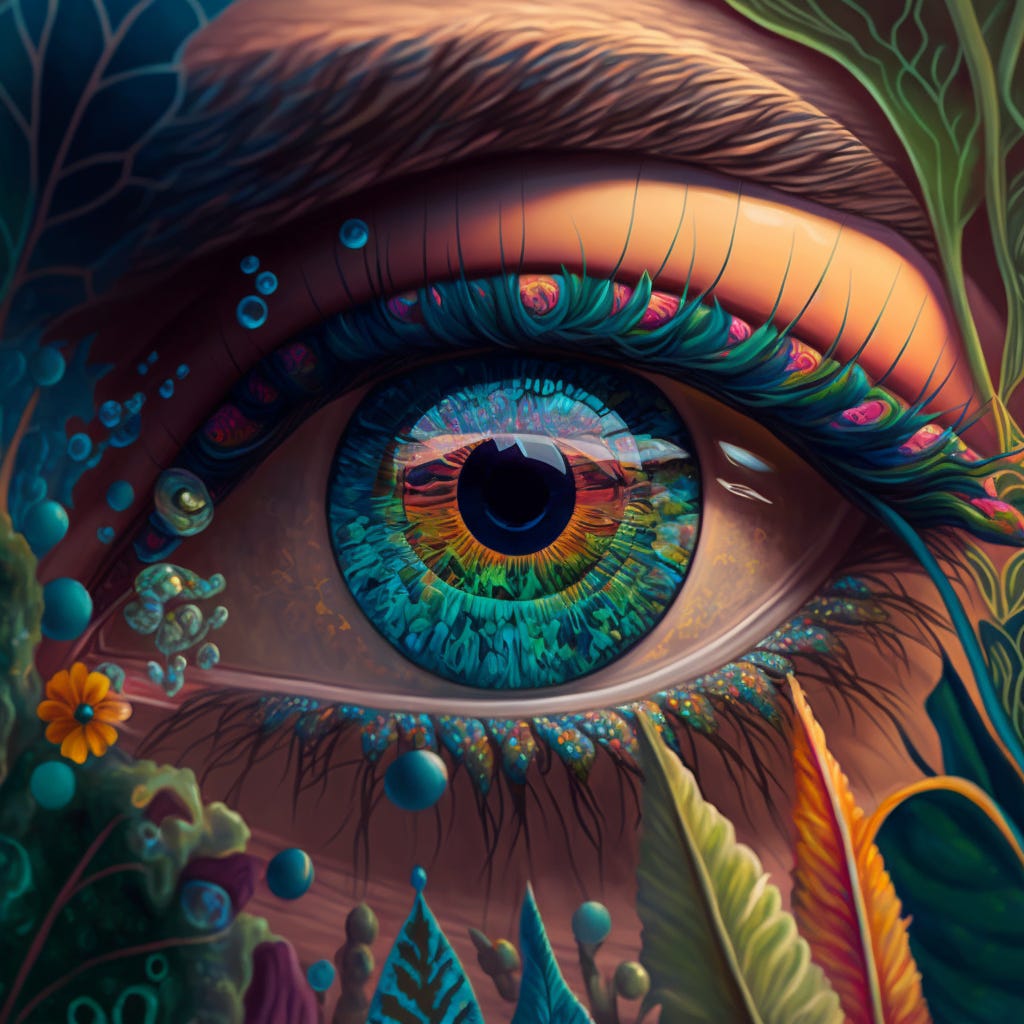The image is an abstract and extravagant piece of graphic art that showcases a close-up of a human eye. The eye is a vibrant mix of colors, including shades of blue, black, green, orange, and intricate patterns in the iris with blues, purples, and reds. The white of the eye is tinged with a yellowish pink hue. Surrounding the eye, the lashes are adorned with various colors and resemble tiny flowers or polka dots on the bottom, while the top lashes appear like green pieces of grass. Above the eye is a prominent eyebrow, adding depth to the piece.

The background and foreground elements add to the complexity of the artwork. On the bottom left and right, there is an array of colorful foliage in psychedelic hues, such as blue, orange, and green, with a distinct yellow flower visible among them. Blue spheres float throughout the image, some of which appear connected to plant-like structures. The upper corners of the image feature large green leaves, framing the eye and adding to the lush, abstract botanical theme. The entire composition is a detailed and vividly colorful exploration of graphic artistry, blending realistic elements with surreal, imaginative details.